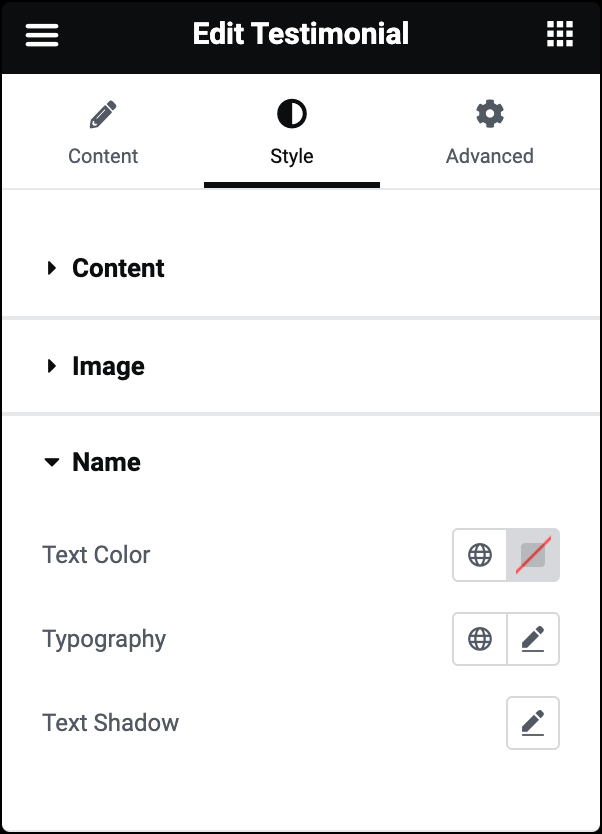This image is a screenshot of a mobile device displaying a settings section titled "Edit Testimonial." At the top of the screen, a horizontal black bar spans the width of the image. In the top-left corner of this bar, there is a button likely used for navigating lists or tabs. Centered at the top is the title "Edit Testimonial," and in the top-right corner, there's a square-shaped button.

Below the black bar, the background transitions to white, with three prominent tabs at the top of this section:
1. **Content** - Indicated by a pencil icon.
2. **Style** - Represented by a half black, half white circle.
3. **Advanced** - Featuring a gear icon.

Beneath these tabs, there are dropdown sections labeled "Content," "Image," and "Name," each presumably containing more options when expanded. Following these dropdowns, the next section includes customizable settings for "Text Color," "Typography," and "Text Shadow." To the right of these settings, there are pencil icons and globe shapes, indicating likely tools for further customization. The final setting in this sequence is solely represented by a pencil icon.